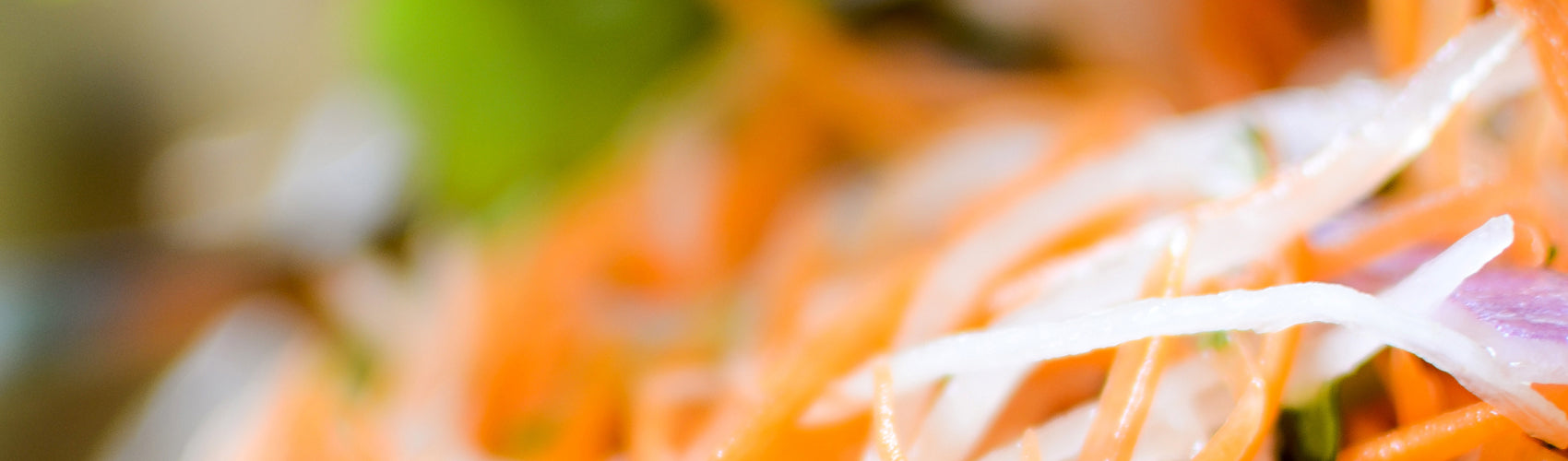The photograph captures a close-up view of a mixed salad with vibrant, shredded vegetables. On the right side of the image, the details are sharp, showing thinly cut, shredded orange carrots with green tips, and finely diced red (or purple) onions. Among the vegetable shreds is a short green stem. Additionally, there are white shreds, likely of radish. The image blurs toward the left, but you can still discern some orange carrots and white shredded vegetables, alongside a vague presence of something green in the background, possibly another type of vegetable. The salad appears to be laid out on a flat surface rather than in a bowl, and the overall composition suggests it could be part of a food preparation process.